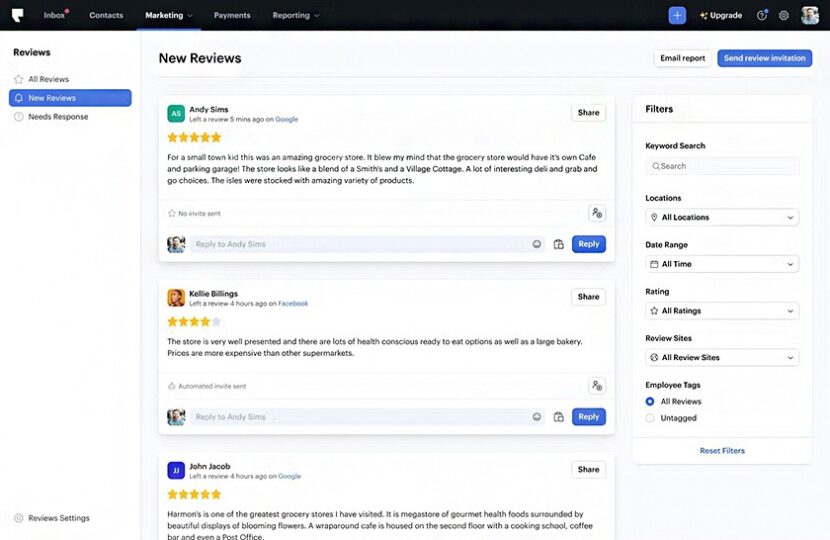The screenshot depicts a reviews page with a white background and a black menu bar at the top. The menu bar contains several sections: Inbox, Contacts, Marketing, Payments, and Reporting. The Marketing section is currently highlighted and active. 

On the right side of the menu bar, there is a blue plus button, an upgrade option, and additional icons including a settings icon. In the far right corner of the menu bar, there is a small avatar image of an individual.

The main body of the page is divided into two primary sections. On the left side, there is a column titled "Reviews" with three options: All Reviews, New Reviews, and Needs Response. The "New Reviews" section is selected, displaying comments from various individuals. Each comment includes a star rating, a brief paragraph of text, and a blue reply button at the bottom. 

On the right side of the screen, there are additional sections for searching and filtering reviews by Filters, Locations, Date Range, Rating, and Employee Tags. At the top corner of this main section, there is a blue button labeled "Send Review Invitation," and next to it, an unhighlighted button labeled "Email Report."